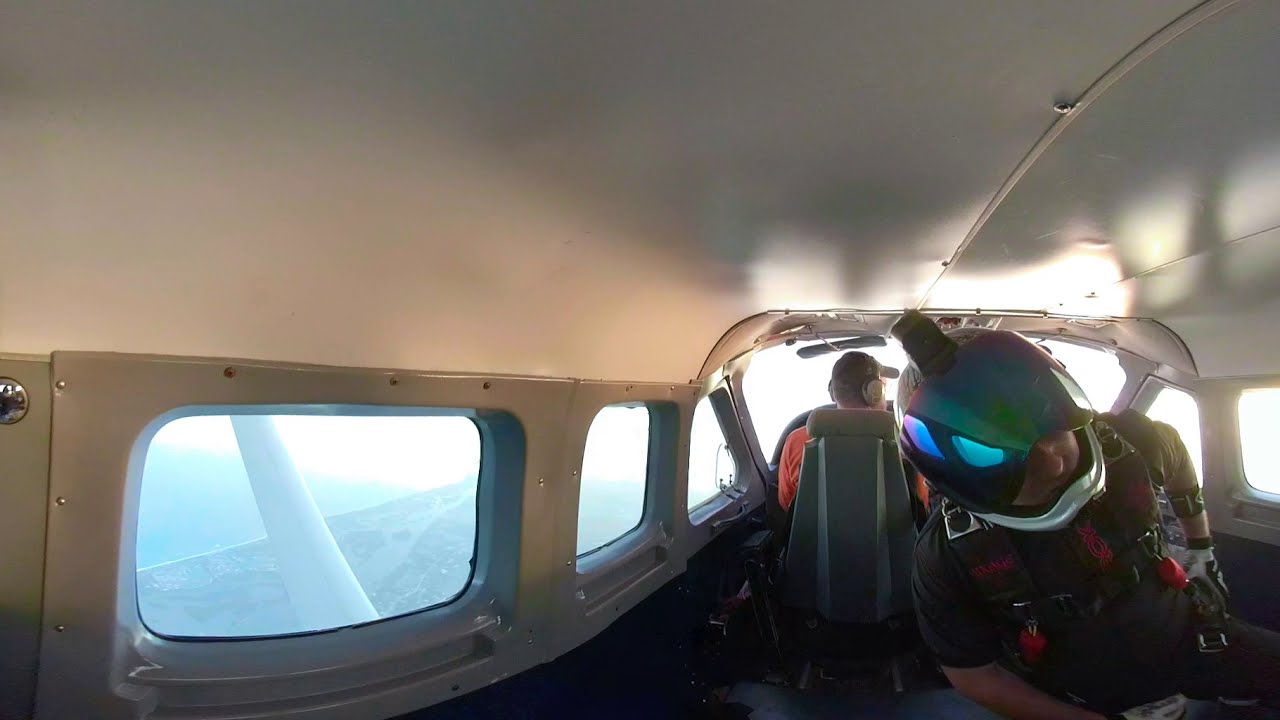This detailed photograph showcases the interior of a small aircraft in mid-flight. In the foreground stands a person facing the camera, adorned in a marbled green, blue, and magenta helmet, indicative of preparing for skydiving, accompanied by black clothing, safety equipment, and gloves. The individual's stance and gear suggest imminent parachuting activities. Seated in front of this person, with his back to the camera, is the pilot, easily identifiable by his orange jacket, baseball cap, and earmuffs, focused on flying the plane. The plane’s metallic interior boasts a white roof and cream-colored walls, with windows that offer glimpses of the wing and a patch of ground far below, hinting at the altitude. The minimalist setup highlights this as a small aircraft, likely suited for just a few passengers.